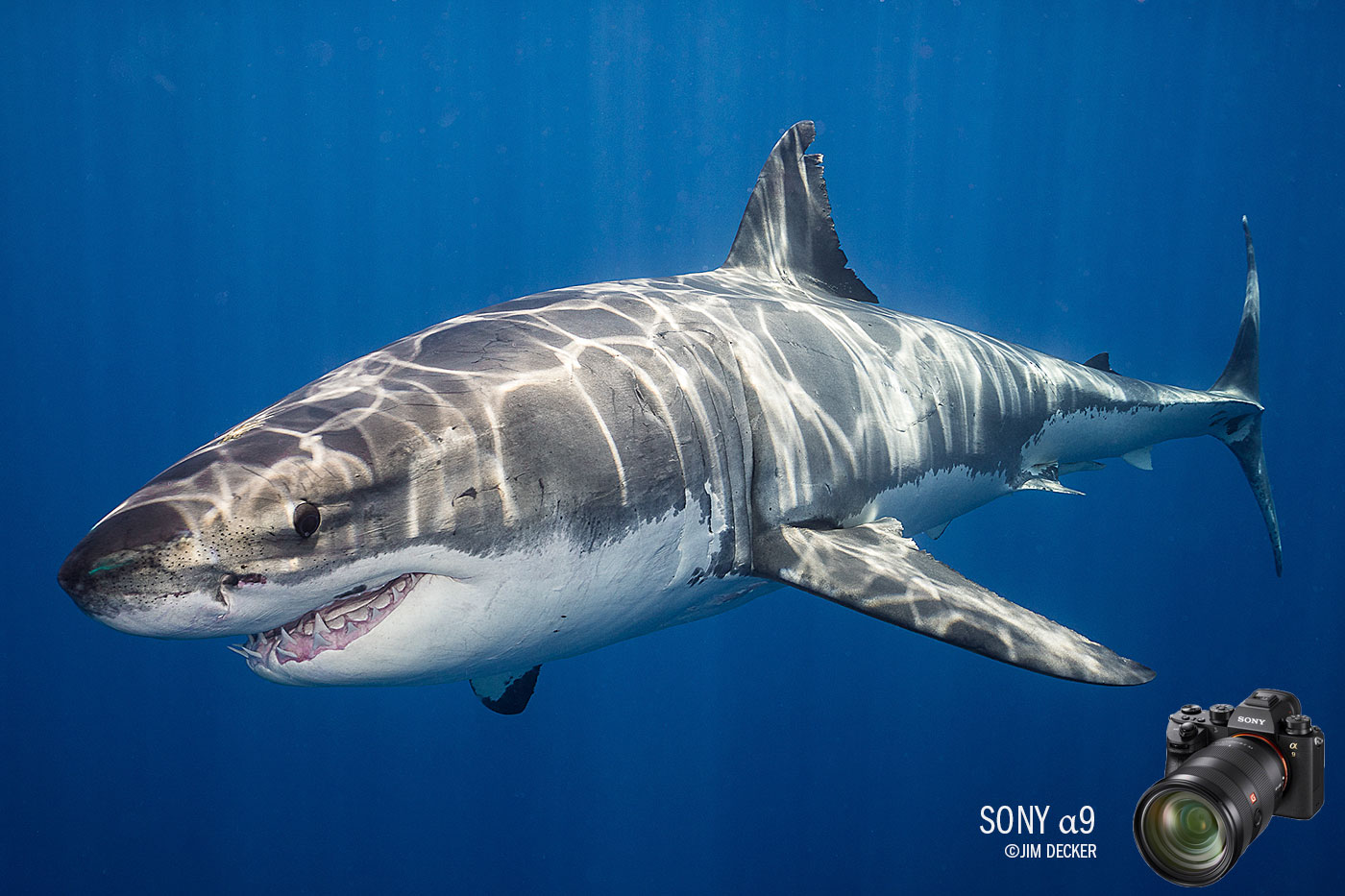This striking underwater photograph captures a powerful shark as it glides through the deep blue sea, positioned prominently at the center of the frame. Light rays penetrate the clear, tropical waters, creating a mesmerizing array of spirals and white lines that dance across the shark's grey skin. These sunlit patterns give the shark's body an intricate, almost ethereal design. The shark is facing left, allowing a clear view of its white underbelly, one dark eye, and a mouth slightly ajar, revealing rows of sharp, pointed teeth. A small nick is visible on its dorsal fin, adding a hint of character to this majestic creature. The image is marked with a subtle overlay in the bottom right corner, where "Sony A9" and "© Jim Decker" are inscribed in white text. Adjacent to the text is an inset image of a black Sony DSLR camera with a zoom lens, suggesting the high-quality photography capabilities of the featured camera.